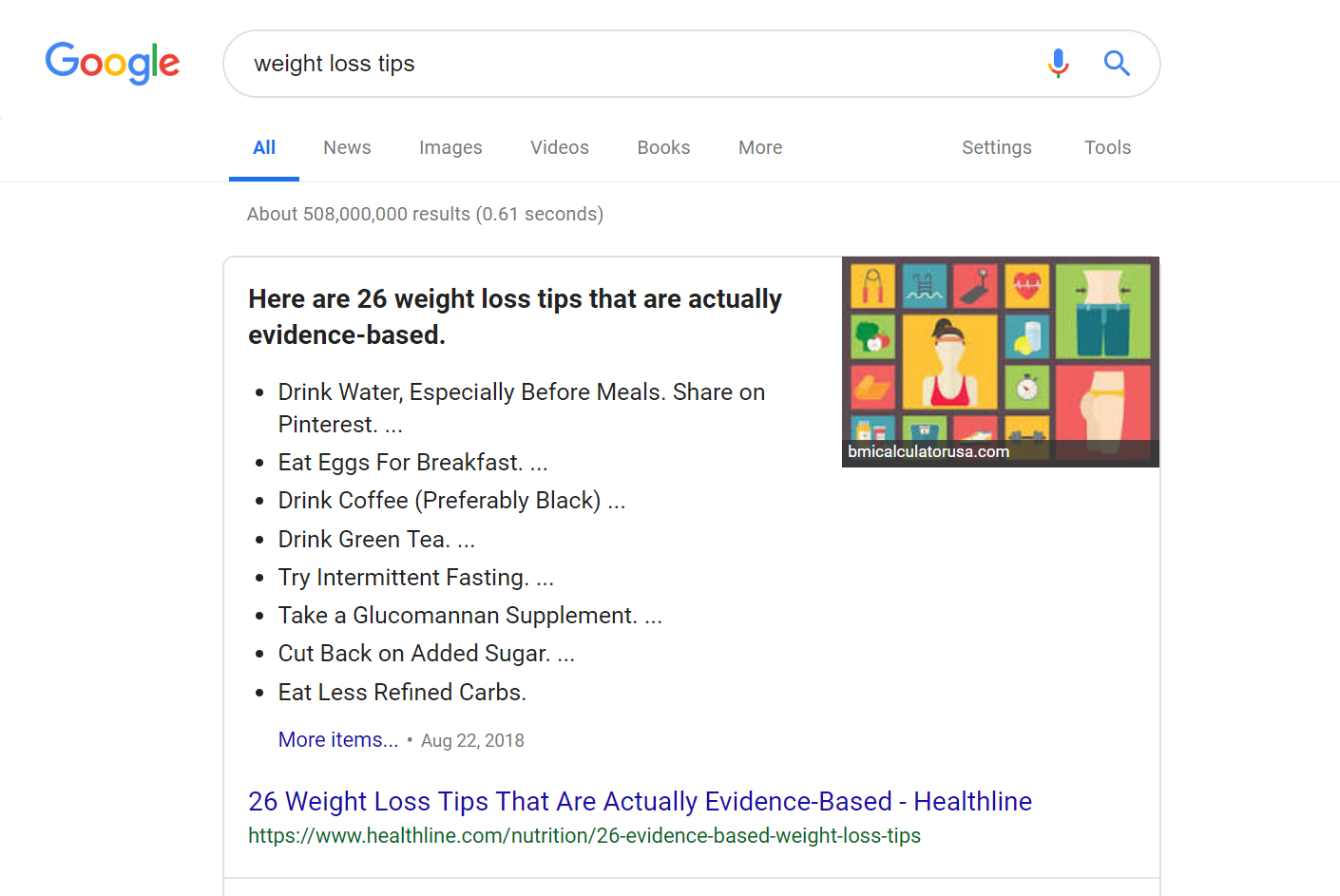This image is a screenshot of a Google search results page. Dominating the top left corner is the iconic Google logo, with its letters brightly colored in blue, red, yellow, and green. Adjacent to the logo is a search bar containing the typed query, "weight loss tips."

Below the search bar, a featured snippet section is prominently displayed. The snippet, titled "Here are 26 weight loss tips that are actually evidence-based," begins with several bullet points:

- Drink water, especially before meals
- Eat eggs for breakfast
- Drink coffee, preferably black
- Drink green tea
- Try intermittent fasting
- Take a glucomannan supplement
- Cut back on added sugar
- Eat less refined carbs

At the end of this list, there is a small blue link labeled "more items," accompanied by the date "August 22nd, 2018."

At the bottom of the image, another blue link reads, "26 weight loss tips that are actually evidence-based helpline," with the URL of the website displayed below it in green text.